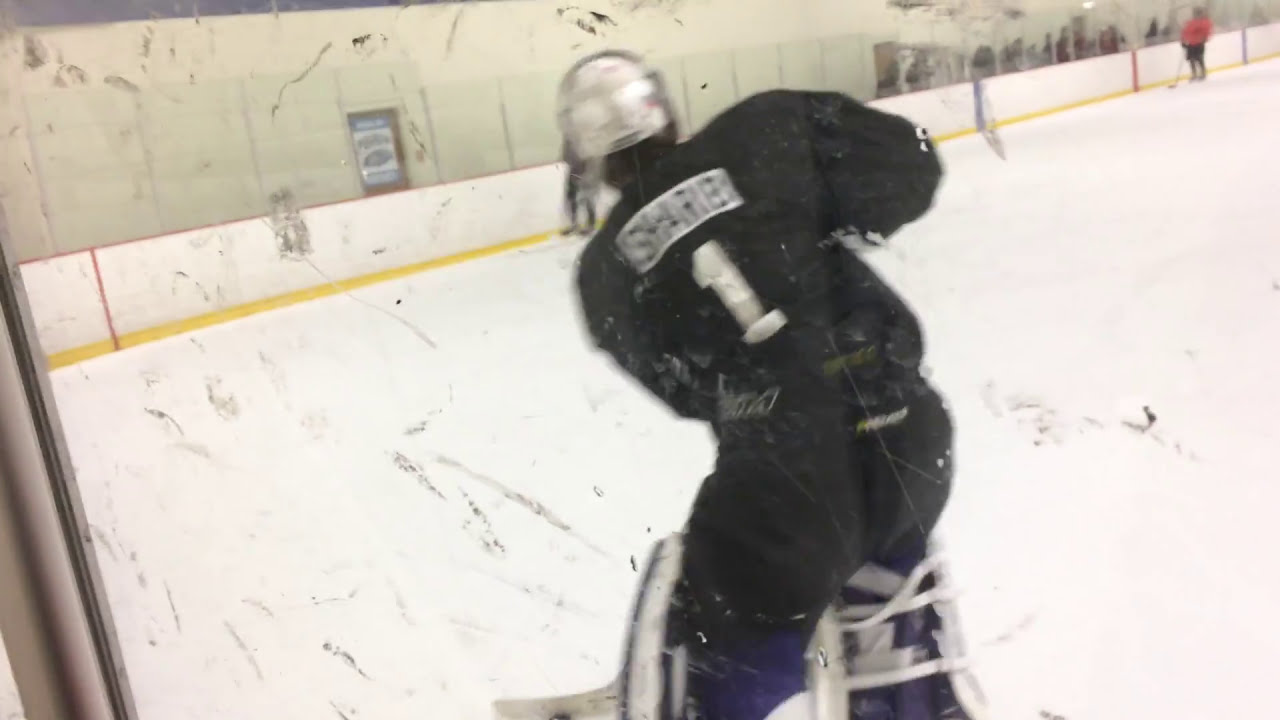The image captures a dynamic scene inside a well-used hockey rink, observed from behind a heavily scuffed safety glass bearing numerous puck marks. Central to the frame is a hockey goalie, dressed predominantly in black with a striking white number '1' emblazoned on his uniform. His name, starting with 'S' and ending with 'B' or possibly resembling 'Asherebe,' is barely legible above the number due to motion blur. The goalie, equipped with prominent leg pads—black with purple and white detailing—and a gray or silver helmet, is captured mid-action, likely moving left and in the process of shooting the puck.

The surrounding rink features white ice, enclosed by boards with a distinctive yellow trim at the bottom and a red trim at the top. In the background, to the left, is a door, while to the right, another player in a red shirt holding a hockey stick is visible. Additionally, pixelated figures, possibly spectators or additional players, can be discerned in the top right part of the image, indicating some crowd presence. The overall scene is a vibrant, albeit slightly blurry, snapshot of an engaging moment in a bustling hockey game.